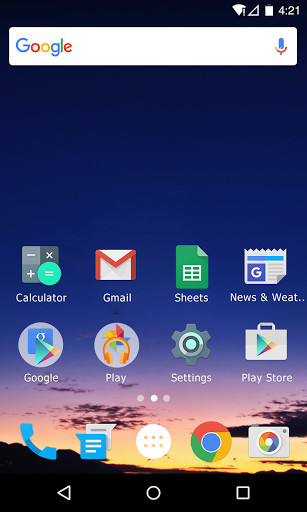A detailed depiction of a smartphone screen captures the essence of a bright, clear day with a blue sky background and scattered clouds. The central element of the screen is a Google search bar, where each letter of "Google" is distinctly colored: blue for 'G,' red for 'o,' yellow for 'o,' blue for 'g,' green for 'l,' and red for 'e.' Adjacent to the search bar is a microphone icon adorned in Google's signature colors for voice search functionality. 

Above this, several app icons are arranged, including a calculator, a chat icon displaying overlapping blue and white speech bubbles, a news and weather widget labeled "W E A T...", and a Google Play Store icon.

Toward the bottom of the screen, there are more interactive elements and application icons. The Google Chrome logo is present, alongside a camera icon, a blue phone icon, another chat icon with blue and white bubbles, and a white circular button with a grid layout symbolizing a menu or app drawer with a 3x2 arrangement of dots.

At the very bottom, navigation icons include a left-facing arrow (back), a circle (home), and a square (recent apps). One of the three horizontal dots is highlighted in white, possibly indicating the active home screen among multiple available pages or screens. The interface elements combine a blend of utility and aesthetics set against a serene sky-themed backdrop.